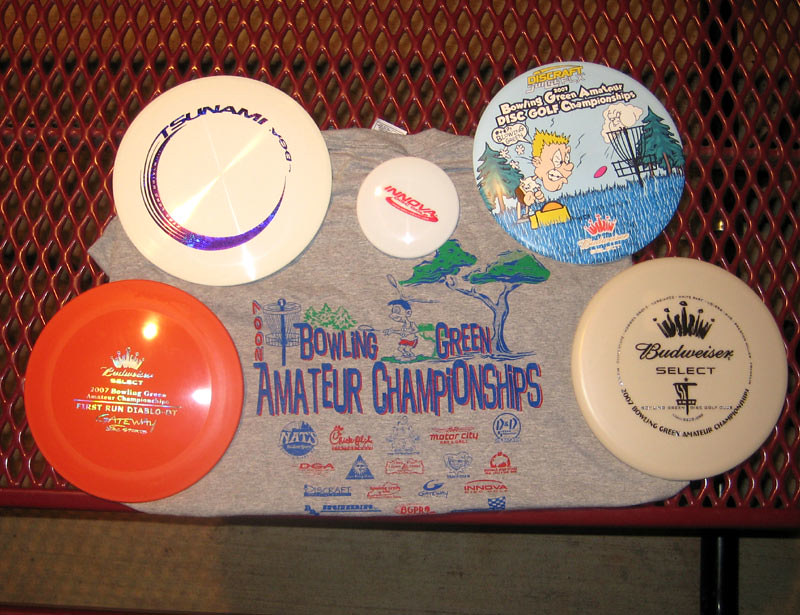This photograph captures a red metal bench with a diamond pattern, typically found in parks, set on a concrete floor. Atop the bench, there is a gray t-shirt that reads "2007 Bowling Green Amateur Championships," accompanied by numerous corporate logos. Surrounding the t-shirt are five frisbee discs, each distinct in size and design. The largest four are regulation-sized, while the fifth is notably smaller. On the top left, a white frisbee with blue text reads "Tsunami." Below it, an orange frisbee bears the Budweiser Select logo in white text. The centered small frisbee has red writing and says "Innova." To the top right, a disc displays the tournament's logo, similar to the cartoon logo on the t-shirt. Finally, at the bottom right, a blue frisbee is decorated with tournament-related imagery. The entire scene vividly showcases the components likely linked to a disc golf tournament, blending the memorabilia with the outdoor setting.